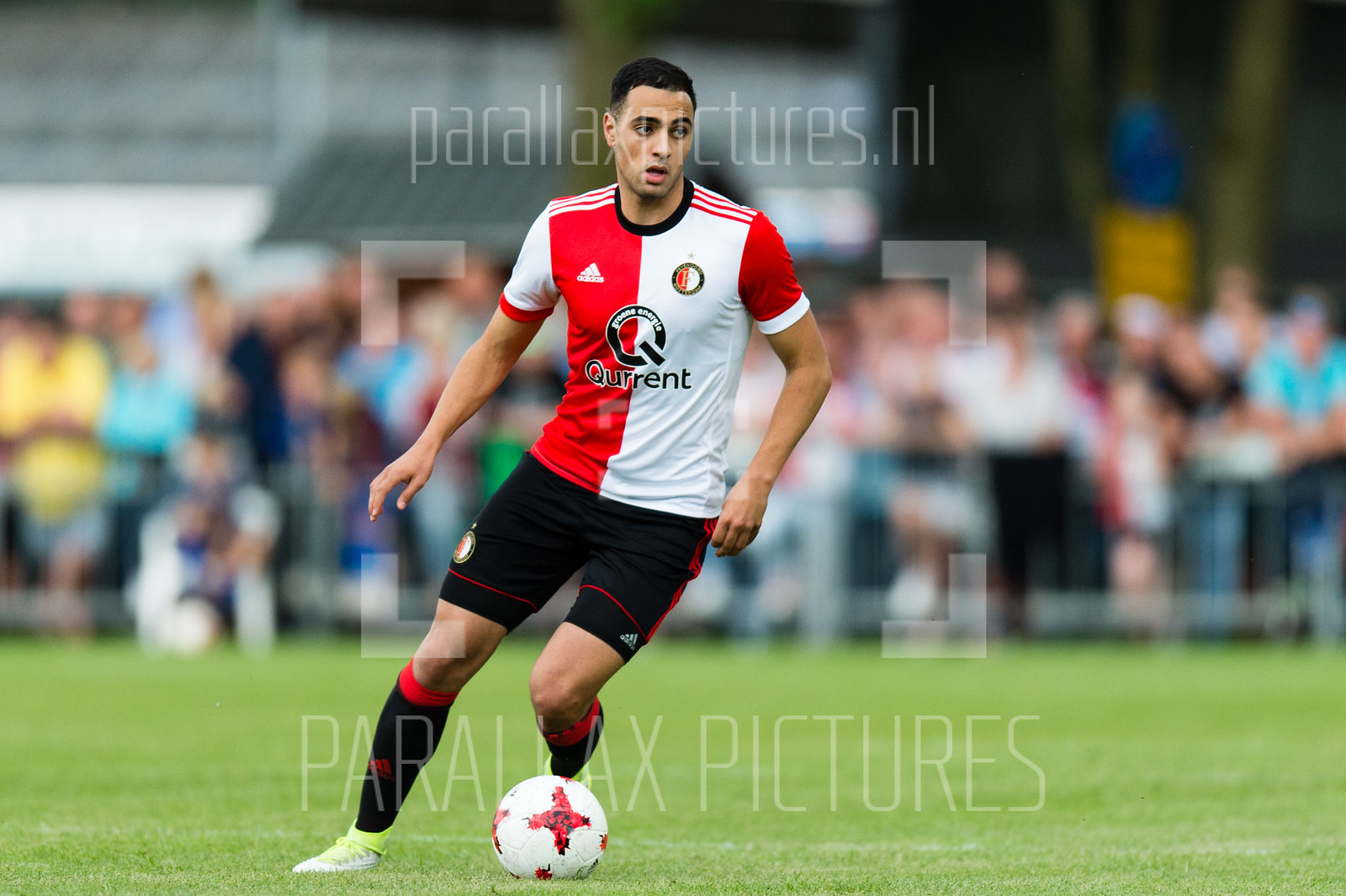The image captures a dynamic moment on a soccer field featuring a soccer player, possibly Hispanic with dark hair, wearing a distinct red and white uniform emblazoned with the word "Corinth." His jersey stands out with its unique design, one half red and white, the other half white and red, complete with the Adidas logo on the red side. He dons black shorts with red accents, black and red socks, and white shoes, all while skillfully kicking a white soccer ball accented with black and red.

The scene is set against a lush green field with a large, blurry crowd of spectators in the background, indicating an intense, well-attended match. Behind this crowd, there are indistinct elements suggesting the presence of a building or trees. Overlaid on the image is a prominent watermark, "parallaxpictures.nl," along with a viewfinder graphic in the center, further branding the photo.